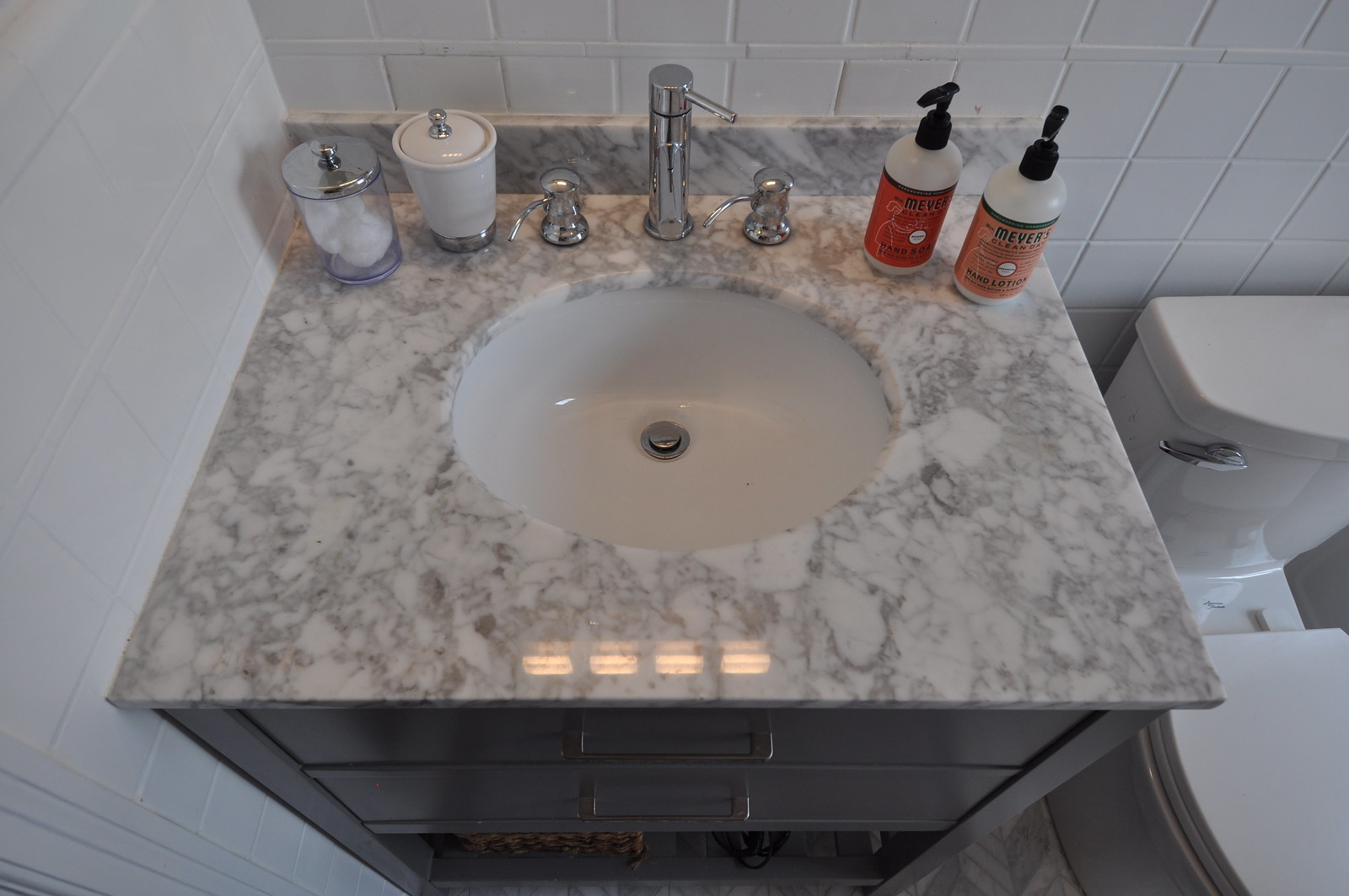A detailed top-down view captures an elegant bathroom setup, featuring a pristine white porcelain wash hand basin. The sink is seamlessly set into a luxurious marble countertop, showcasing an exquisite pattern of white and gray swirls and blotches. Below the basin, there is a dark wood cabinet with two drawers, adding a touch of warmth and contrast to the space. On the left side of the polished chrome faucet sits a collection of personal care containers, while on the right, two stylish bottles of Myers hand soap are neatly arranged. The backdrop features white square-tiled walls that enhance the room's clean and modern aesthetic. To the right of the sink, a white toilet with the seat lowered adds to the cohesive look of this meticulously designed bathroom.